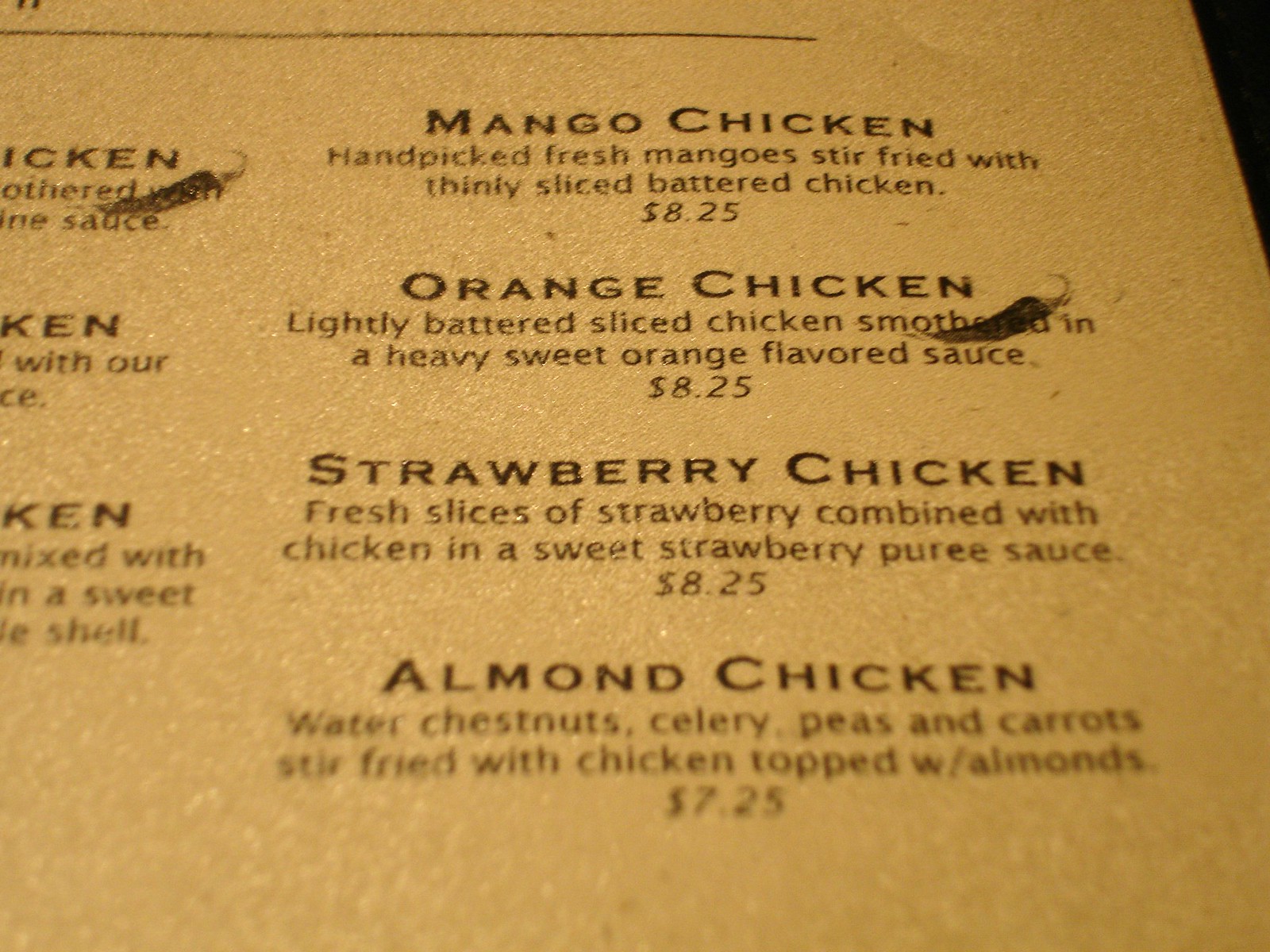The image depicts a section of a parchment-like menu with a brownish-gold hue, adorned with elegant calligraphy. The menu appears to be divided by thin horizontal lines, and features dish names in bold capital letters, followed by descriptions in mixed-case text. Each item is priced, and there are periodic punctuation marks used consistently across the menu.

At the top, the menu lists:

1. **MANGO CHICKEN**
   *Hand-picked fresh mangoes stir-fried with thinly-sliced battered chicken. $8.25.*

   Following Mango Chicken is:

2. **ORANGE CHICKEN**
   *Lightly battered sliced chicken smothered in a heavy sweet orange-flavored sauce. $8.25.*

3. **STRAWBERRY CHICKEN**
   *Fresh slices of strawberry combined with chicken in a sweet strawberry puree sauce. $8.25.*

And finally:

4. **ALMOND CHICKEN**
   *Water chestnuts, celery, peas, and carrots stir-fried with chicken topped with almonds. $7.25.*

Additionally, there are two symmetrical splotches on the menu, one partially obscuring the word "smothered" under the Orange Chicken description and the other positioned on the left side. These splotches resemble small carrots with tops, although their exact nature is unclear.